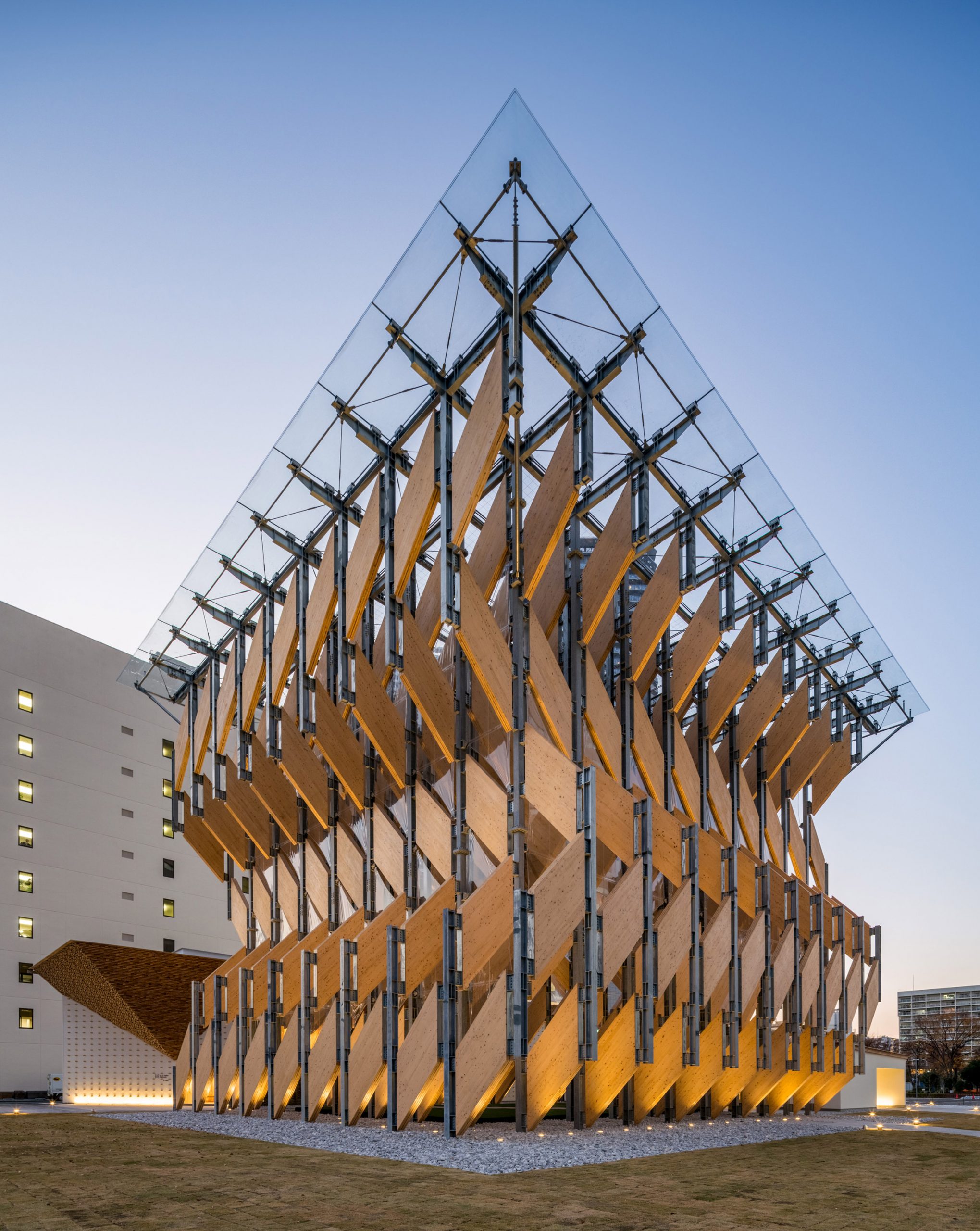The image depicts a striking outdoor sculpture that stands nearly as tall as the multi-story white building behind it. The structure features a series of trapezoid-shaped wooden slats in various shades of yellow, tan, and darker stains, arranged in detailed, criss-cross patterns reminiscent of argyle. These wooden panels are intricately mounted on vertical gray metal rods that form an X-shaped frame. Above, a clear glass roof tops the structure, offering a striking contrast to the earthy tones of the wood. This modern, architecturally impressive piece is set atop a gravel-covered platform amidst an open sky, with additional smaller buildings visible in the background.